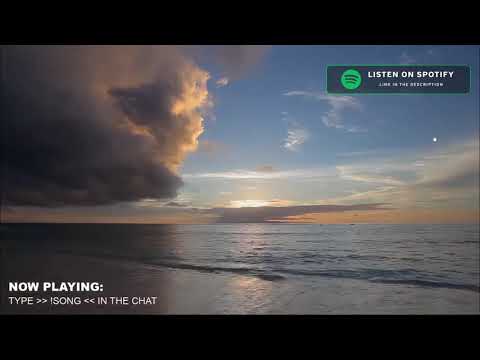The image is a serene beach scene, resembling an album cover, promoting a song on Spotify. It captures a tranquil seascape at sunset with calm, blue waters meeting beautiful brown sand. The sky is a stunning mix of blue, orange, and white, featuring wispy clouds tinged with the glow of the setting sun. A hint of moonlight begins to emerge, adding a unique touch to the scene. In the bottom left corner, there's text indicating the song now playing with a prompt saying "type iSong in the chat." In the top right corner, the Spotify logo and text instruct to "listen on Spotify." The dreamy landscape, with minimal waves and a gentle blend of colors, evokes a peaceful, almost magical ambiance.